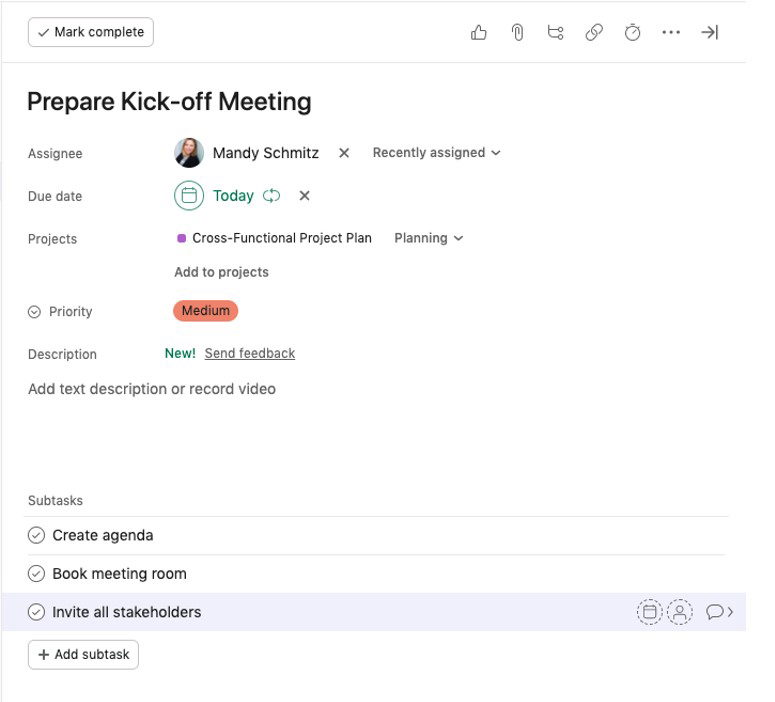**Detailed Task Overview for Project Kick-Off**

The image represents a task management interface for a project kick-off meeting. 

- **Header Section**:
  - In the upper left corner, there is a button labeled "Mark Complete" with a checkmark icon.
  
- **Right Side Icons**:
  - Thumbs up
  - Paperclip (attachment)
  - Thought bubble
  - Share
  - Two overlapping ovals
  - Clock
  - Three dots and a line
  - Arrow pointing to a vertical line

- **Main Task Details**:
  - The largest font reads "Prepare to Kick Off Meeting," written in black on a white background.
  - The assignee for this task is Mandy Schmitz, indicated by the text "Assignee: Mandy Schmitz" with a small 'X' next to her name, signifying that it is recently assigned.
  - Dropdown options include:
    - **Due Date**: Today (highlighted in green) next to a calendar icon.
    - **Project**: Cross Functional Project Plan (illustrated with an oval containing arrows and an 'X'). The project phase is identified as "Planning" with a dropdown for further options.
    - **Add to Projects**: Button available for assigning the task to additional projects.
  - **Priority**: Set to medium, identified by a red button.
  - **Description**: Indicated as new, marked by a green label.
  - **Send Feedback**: Underlined text, offering an option to submit feedback.

- **Subtasks**:
  - Subtasks are listed with bullet points, each marked by a circle containing a checkmark. These subtasks include:
    - Create an agenda
    - Book a meeting room
    - Invite all stakeholders

  Below these items, there is a button labeled "Add Subtasks," allowing for the inclusion of additional subtasks.

This detailed structure ensures clear communication of the preparation steps and tools necessary for the efficient execution of the project kick-off meeting.